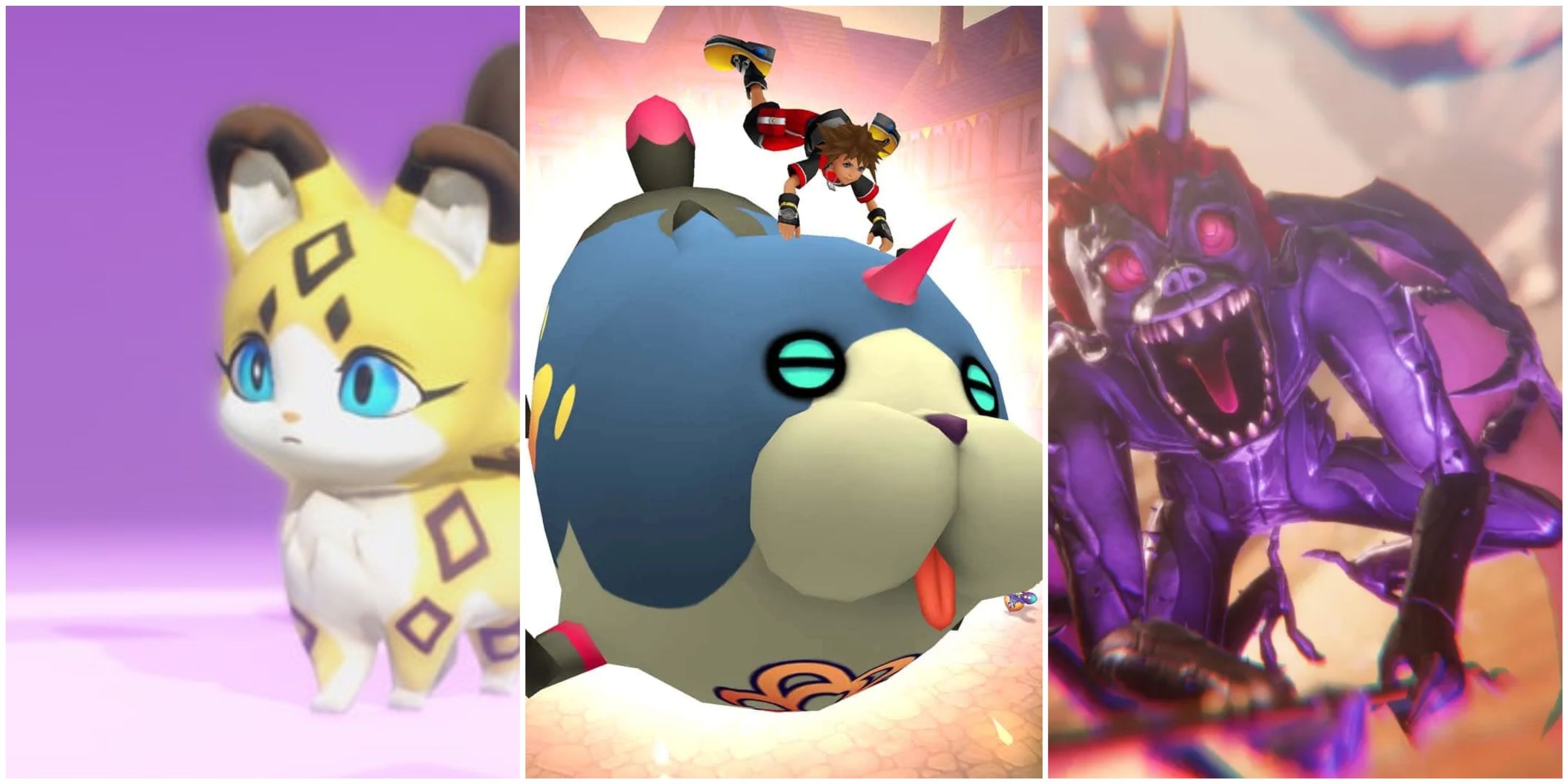This image showcases three side-by-side animated characters, each set against a distinct background within equally-sized rectangles. The leftmost image features a cute, cartoonish yellow cat with big blue eyes, a white belly, and white fur around its mouth area and inside its ears, which have brown tips. The cat also has purple diamonds on its sides and a black diamond on its forehead, set against a purple background with a light purple floor.

The center image displays a large, puffy creature resembling a dog with a blue top and a white bottom. It has a pink horn on its head and glowing neon blue eyes with black lines. Additionally, its tail is black with a pink tip. A boy is seen hanging onto its back, seemingly riding the creature, with an impression of an explosion in the background.

In the rightmost image, there is a menacing robotic bat-like demon, squatting with a wide-open mouth full of sharp teeth. It has purple horns, red hair, and glowing pink eyes, complemented by long, spiky feet and forward-flapping wings, suggesting it is about to take flight. The character exudes an ominous presence, contrasting sharply with the more innocent leftmost image.